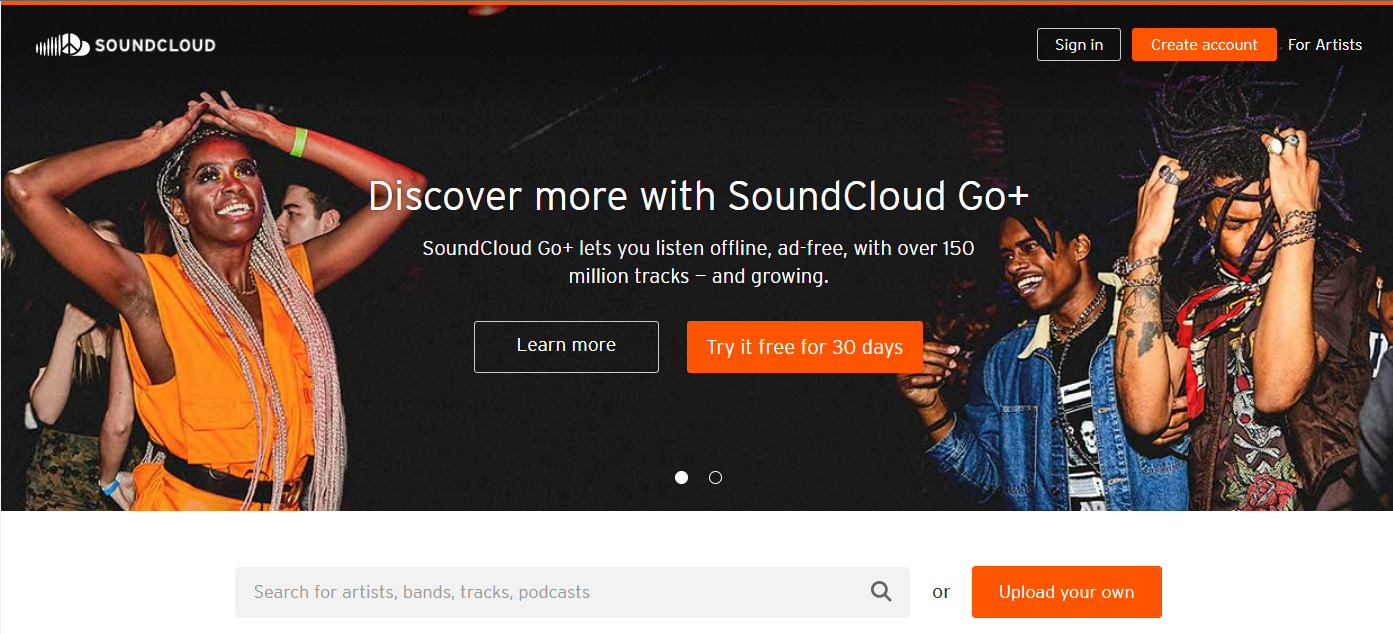The screenshot features a black background. In the upper left-hand corner, there is a prominent white SoundCloud logo. Positioned to the right of the logo is the word "SOUNDCLOUD" in bold, white, all-caps. On the upper-right side of the image, three distinct buttons are displayed: a black sign-in button outlined in white with the text "Sign-In" in white, an orange "Create Account" button with white text, and another black button that says "For Artists" in white.

In the center of the image, about six lines down, bold white text proclaims, "DISCOVER MORE WITH SOUNDCLOUD GO+". Two lines below, another block of white text provides additional information: "SoundCloud Go+ lets you listen offline, ad-free, with over 150 million tracks—and growing."

Below this descriptive text, two large buttons are centered: a black "Learn More" button with white text on the left, and an orange "Try it for free for 30 days" button, also with white text, on the right.

To the left of these buttons is an image featuring a dancing black woman. To the right of her, a couple is seen dancing. Below this image, there is a notable white space followed by a gray search bar. To the right of the search bar, small black text that states "or", and an adjacent orange rectangle with the text "Upload your own" in white completes the interface elements.